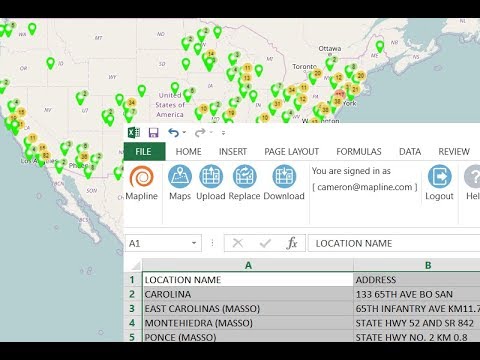This screenshot shows a detailed map primarily featuring the United States, with portions of Canada visible as well. The map is adorned with a multitude of green markers scattered across various locations, with significant clusters in some areas and sparse distribution in the upper left and upper right sections. Additionally, yellow circles containing numbers are interspersed on the map, indicating specific data points or locations. The body of water depicted on the map is rendered in a grayish-blue hue, providing a contrasting backdrop to the landmasses.

At the top and bottom of the page, there are black bars framing the image. Dominating the lower section of the image, a pop-up screen obscures a considerable portion of the map. This screen displays a list of location names and addresses, suggesting detailed information about the mapped points. Above the pop-up, interface tabs are visible, labeled "File," "Home," "Insert," "Page Layout," "Formulas," "Data," and "Review," indicating an interactive, likely software-based environment.